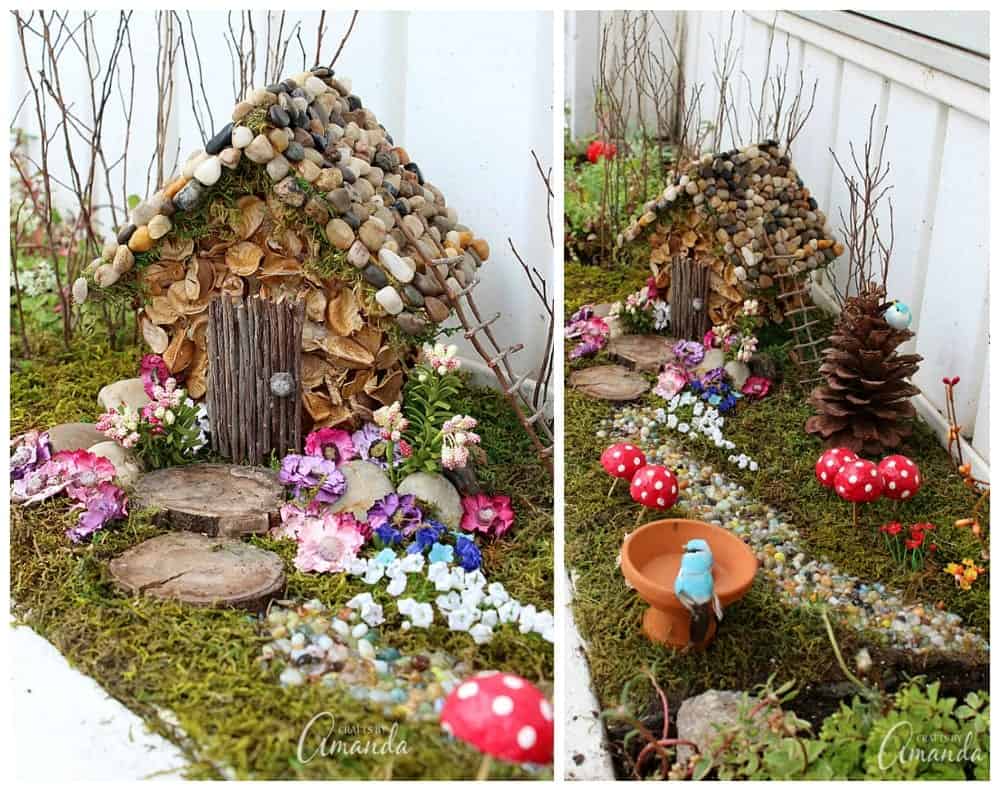In this captivating outdoor scene, there are two photographs showcasing a meticulously crafted miniature house, standing approximately 6 inches tall, constructed from natural materials. The house features a roof made of rocks, walls fashioned from leaves, grass, and cedar chips, and a charming door built from tiny broken twigs. A little stone serves as a door handle. The right-side image provides a frontal view of the structure, highlighting a quaint ladder leading up to the roof. At the front entrance, two wooden discs create a walkway that transitions into a meandering path crafted from small stones, which curves down and to the right, accentuated by tiny mushrooms and vibrant flowers. A pine cone stands nearby, mimicking a tree, and there's an inventive bird feeder with a little blue bird resting on it at the bottom left of the screen. The second photo offers a different angle, revealing additional details like the birdbath and the surrounding greenery. The entire setup evokes a whimsical fairy tale or gnome garden feel, nestled comfortably in a lush, natural setting.